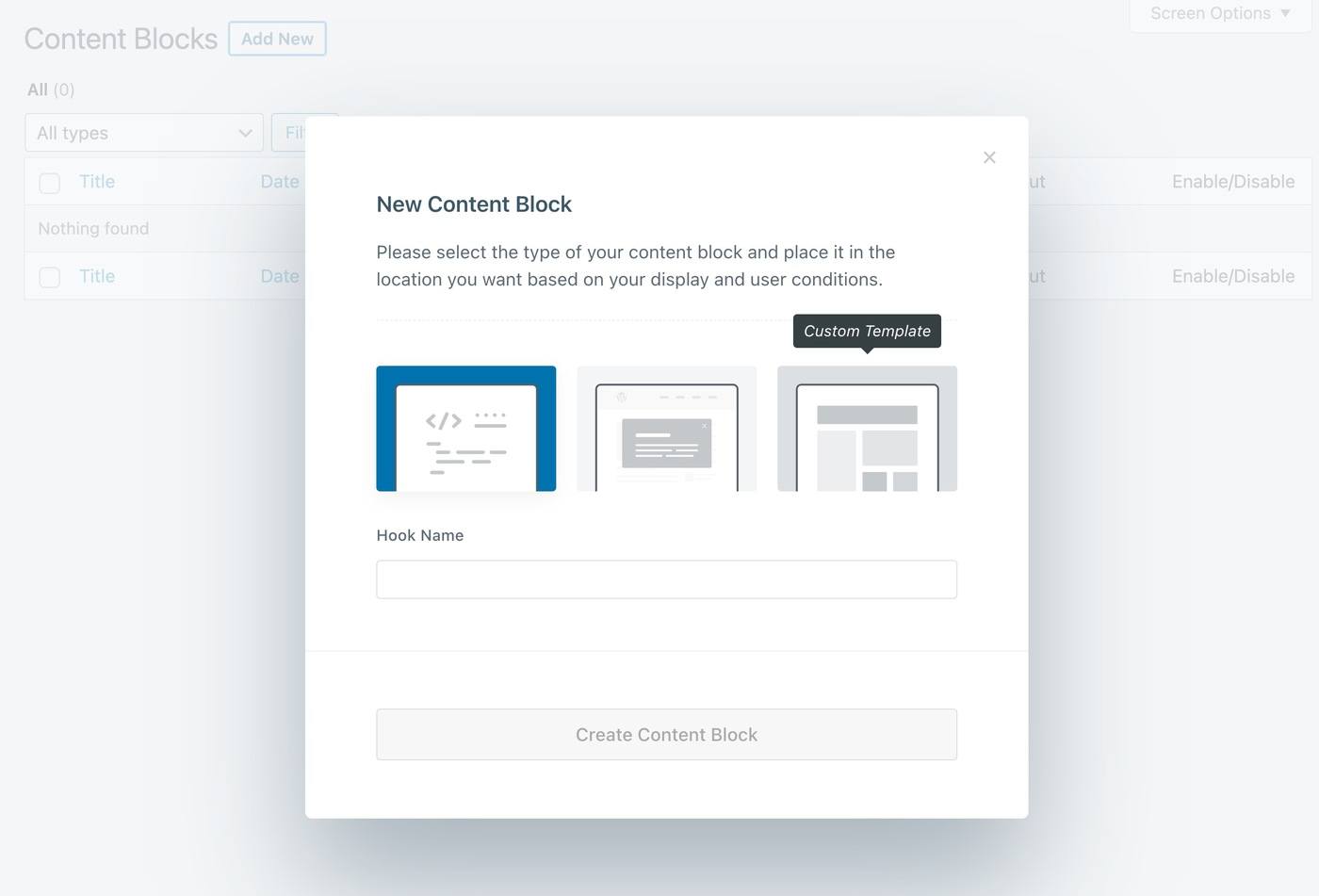This image depicts a website interface for managing content blocks. In the upper left corner, a section titled "Content Blocks" features a prominent "Add New" button displayed in a blue box. Below this, there are filter options labeled "All" and "All Types." An area designated for titles, marked in blue, indicates that "Nothing Found" under the current search or filter criteria.

The entire view has a semi-transparent overlay that obscures full readability, showing only dim shadows and partial text. On the top right corner of the interface, there are options labeled "Screen Options," which include toggles for "Enable" and "Disable."

A pop-up window is also visible, titled "New Content Block." This window instructs users to "Please select the type of your content block and place it in the location you want based on your display and user conditions." It features multiple icons representing different device types; the first one, which resembles an iPad, is outlined in thick blue, indicating it is selected. The second icon has a gray outline, while the third, labeled "Custom Template" in black text, also has a gray outline.

Further down in the pop-up, there is a field labeled "Hook Name" with an empty input box. Beneath this input box, the option to "Create Content Block" is presented inside a shaded gray box, indicating it is a clickable button.

Overall, the interface appears designed to help users easily create and manage various content blocks tailored for different devices and templates.